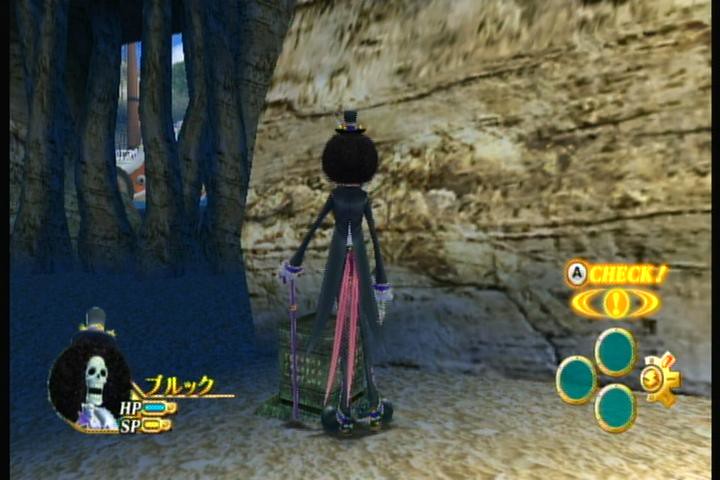In this video game screenshot, a tall, thin character stands with their back to the camera, depicted against a diverse, richly detailed background. The figure has a round, bulbous head, black in color, and is whimsically adorned with a tiny, undersized top hat. Encircling their neck is a set of white ruffles, adding a formal touch to their dark, sophisticated attire. They wear a black coat featuring a V-shaped back and striking red tails, accompanied by black pants and shoes.

The character's hands are clad in white gloves, with one hand gripping a purple cane, completing their elegant, somewhat mysterious look. They stand on a tan, sandy ground beside a dark, textured rock wall which provides a stark contrast to the bright, open space. In the background, large, thick, and very dark tree trunks shoot upwards, adding depth and an almost foreboding atmosphere to the scene.

To the left of the character, there's a skeleton with hit point and power indicators, which suggests impending action or combat. On the right side of the image, three turquoise dots encircled in gold and a gold design resembling a four-point keypad add to the interface elements of the game. Above these elements, there's a gold circle, further contributing to the in-game graphical display. The overall scene is richly textured and captures a moment thick with atmosphere and anticipation.